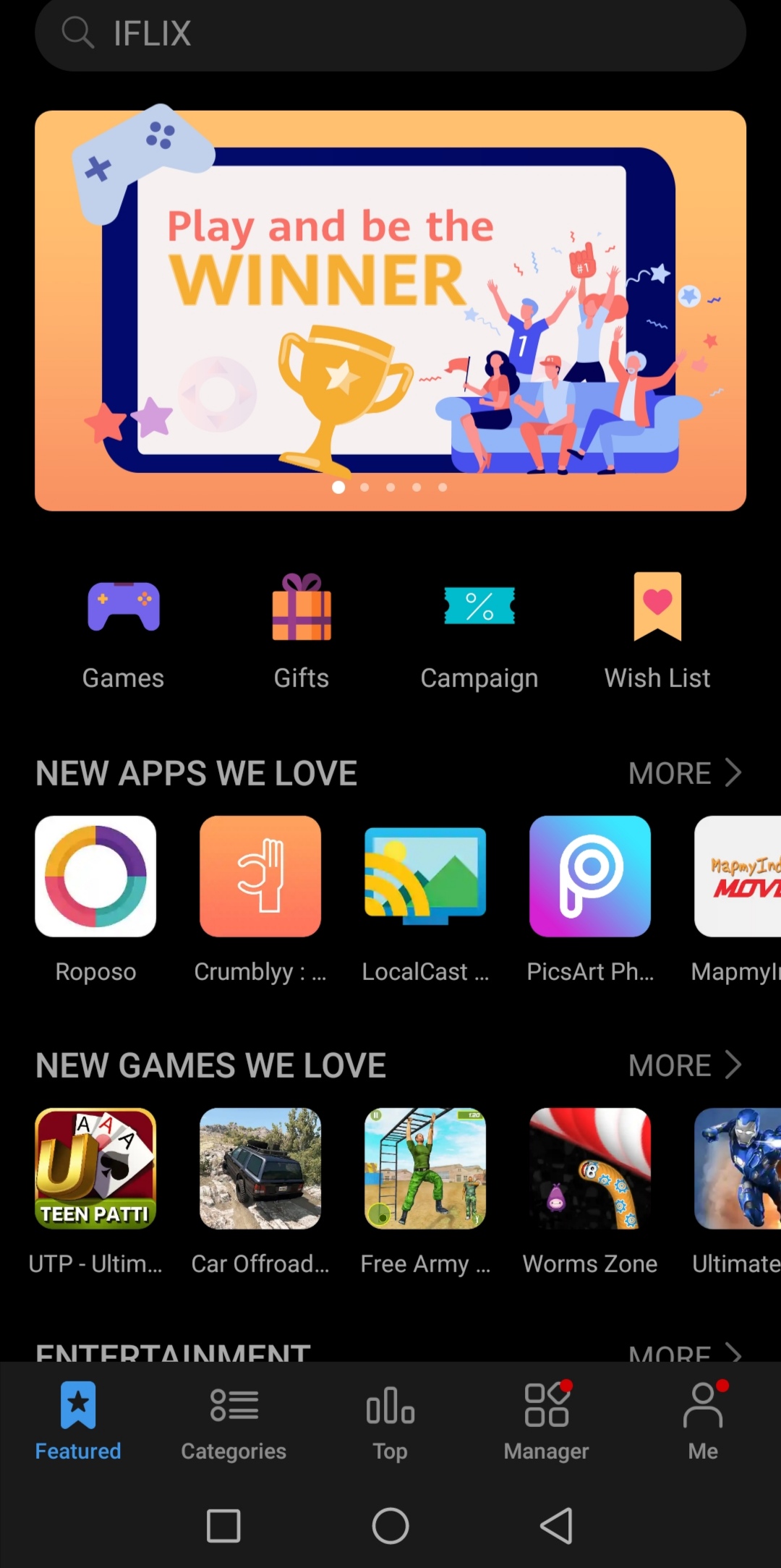Screenshot from the iFlex Company Interface

At the top, a search bar is prominently displayed for easy navigation. Below it, an orange rectangle features the slogan "Play and Be the Winner," accompanied by a cartoon illustration of several people sitting on a couch playing a video game, along with a cartoon award cup.

Four interactive categories are listed immediately beneath: 
1. Games
2. Gifts
3. Campaign
4. Wish List

The section titled "New Apps We Love" follows, showcasing a variety of apps with visually distinct icons:
- "Repozo" – represented by a multi-colored circle
- "Crumbly" – illustrated with an orange finger
- "Local Cast" – featuring a scenery picture with a yellow, rainbow-like shape
- "PixArt" – depicted with a target symbol and a droplet
- "MapMy..." – title partially obscured, written in red font

A further section displays "New Games We Love", including:
- "Teen Patty UTP"
- "Car Off-Road" – featuring an image of a car
- "Free Army" – showing a man performing an overhead workout
- "Worm Zone" – with part of an American flag
- "Metal Gear Ultimate" – depicting a soldier

At the bottom of the interface, a footer provides navigation buttons for further exploration: 
- Featured
- Categories
- Top
- Manager
- Me

Overall, the screenshot presents a vibrant, user-friendly interface aimed at engaging users with a variety of entertainment and app choices.